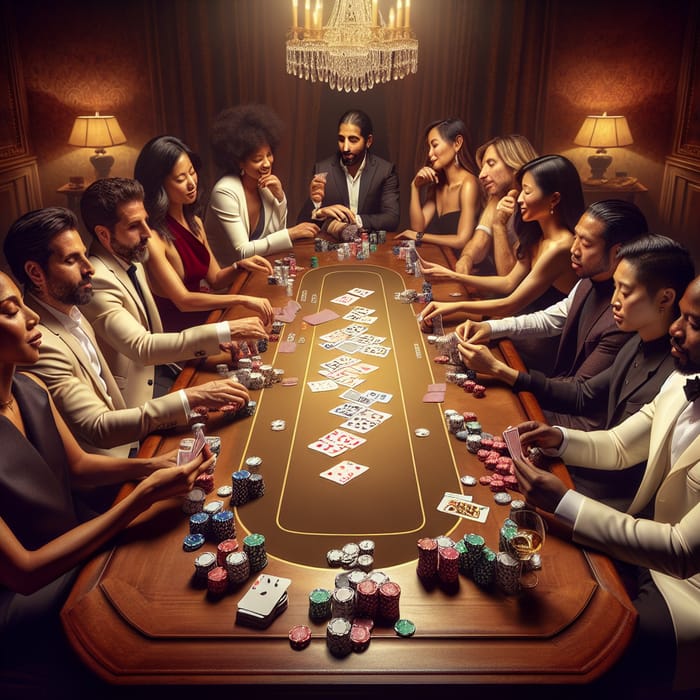In this opulent indoor setting, likely within a well-to-do residence or an exclusive club, a group of men and women gather around a sophisticated wooden table with a brown inset. Scattered across the table is a vibrant array of multi-colored betting chips and an unfamiliar card game involving a long rectangular section down the center, filled with various playing cards. Notably, two nearly identical men, possibly twins, are positioned on the right side, each sporting similar haircuts, mustaches, beards, and immaculate white suits. The room is illuminated by an elegant chandelier hanging above the table and two table lamps situated against the back wall. At the head of the table sits a distinguished gentleman, potentially the host of the gathering.